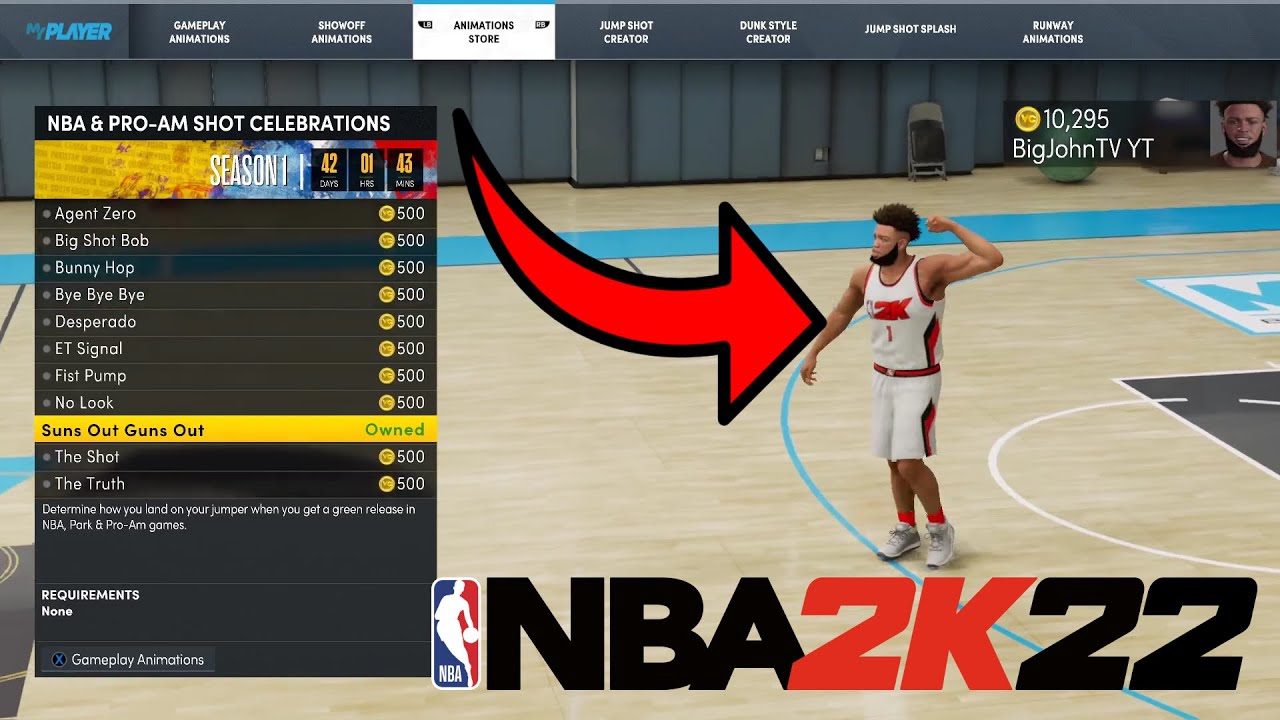In the top left corner, there is a blue logo featuring the word "my" in dark blue, blocky lettering. Following it, in light blue capital letters within the same block-like, italicized font, is the word "player." To the right, there's a menu set against a bluish-gray background. The menu items, displayed in white text, include "Gameplay Animations," "Show Off Animations," "Animation Store," which is currently selected and thus has white text on a black background, "Jump Shot Creator," "Dunk Style Creator," "Jump Shot Splash," and "Runway Animations."

Below this menu, there's a rectangular list of animation names in white text. The first item is "Agent Zero," accompanied by a coin symbol and the number 500. Next is "Big Shop Bob," also valuing at 500 coins. Following are "Bunny Hop," "Bye Bye Bye," "Desperado," and "ET Signal." "Fist Bump," "No Look," and "Suns Out, Guns Out" come next, with "Suns Out, Guns Out" highlighted in yellow, rendered in bold black text, and marked as "Owned" in green lettering towards the right. Below this highlight are "The Shot" and "The Truth," both in standard white text.

On the right side of the screen, there is an arrow pointing to a man in an NBA outfit. He has one arm raised. His uniforms are predominantly white with black and red borders around the sleeves. The sides of his outfit feature a diamond-shaped design with a black border and a red center. He is wearing red socks and white shoes. At the bottom of the image, the NBA 2K22 logo is visible.